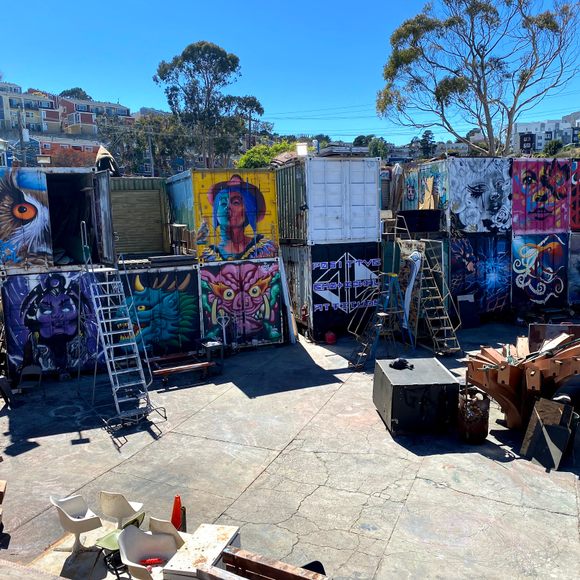The image depicts a vibrant, outdoor setting featuring twelve large steel shipping containers, stacked in a formation of six rows with two containers per row. These containers serve as a canvas for a series of professionally painted murals, showcasing diverse subjects such as an owl, a pop art lady, a dragon face, and various animal heads. Prominently, a striking mural of an African American woman with an Afro contrasts with colorful depictions, including a whimsical monster. Beneath a clear blue sky punctuated by a couple of trees, the scene includes a concrete surface in the foreground. A small seating area with white chairs is visible to the left, beside a black table accompanied by some wood on the right. There are little ladders and built ledges providing access to the upper containers, enhancing the layered aesthetic of this artistic installation. In the background, buildings can be seen, adding depth to the vivid urban tableau.